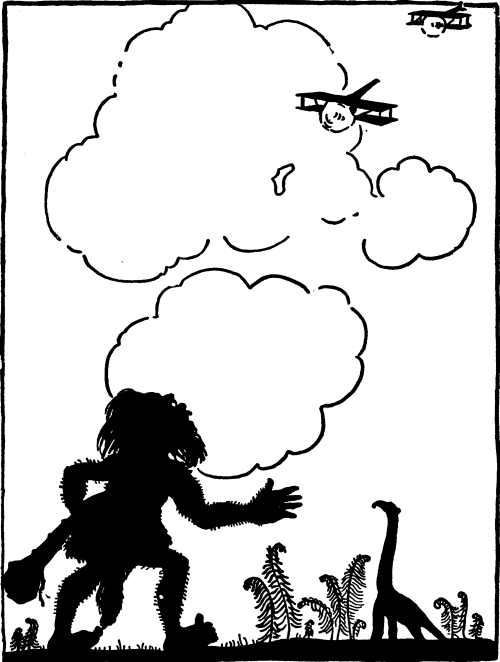In this detailed black-and-white illustration, a humorous scene unfolds featuring a caveman with long, wild hair and big feet, his back facing the viewer. The caveman is depicted holding a club-like tool, with lines indicating body hair and simple clothing. His large toes, particularly his big toe, are distinctly outlined. Next to him stands a prehistoric, long-necked dinosaur among silhouettes of several leafy plants. The entire scene, rendered in solid black silhouettes, is set against a stark white background. In the sky above, suggested outlines of clouds frame two primitive Wright brothers-style airplanes flying towards the caveman and dinosaur, emphasizing the anachronism and adding a comedic touch to the illustration.